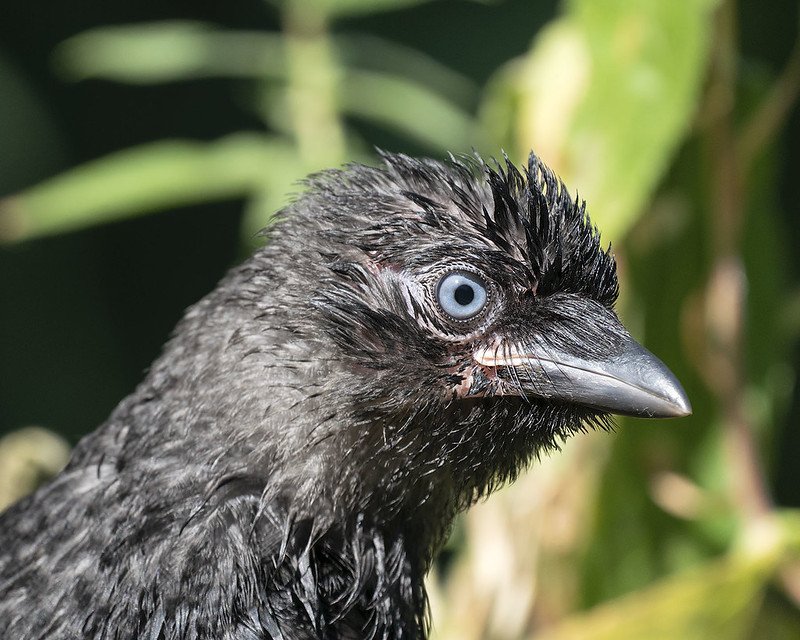This is a tightly cropped, well-lit color photograph of a black bird's head and neck in sharp focus, with the bird facing to the right in profile. The black feathers on its head appear wet, standing in small, spiky formations and revealing hints of the pink skin underneath. The bird's eye is a striking light blue with a deep black pupil, capturing attention as the main focal point. The black beak is closed. The background consists of indistinct green foliage, blurred to emphasize the bird's detailed feathering and features. The sunlight enhances the minutiae and sheen of the wet feathers, adding to the clarity and vividness of the image.